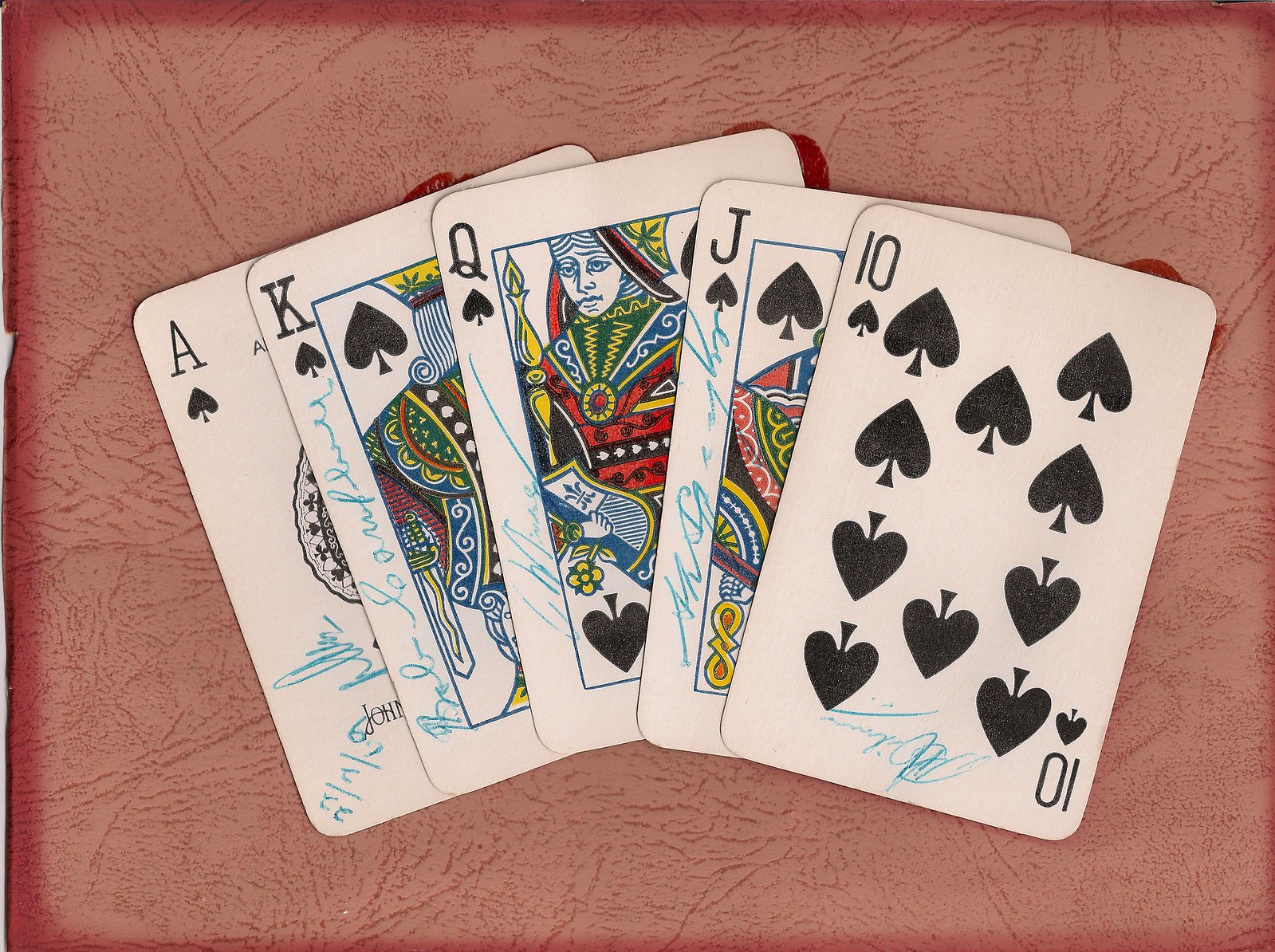A hand of poker showcases a remarkable Royal Flush comprising an Ace, King, Queen, Jack, and Ten, all in spades. Each card bears multiple signatures in blue ink, written in cursive by various individuals, signifying a possible celebration of this rare occurrence. The cards follow the traditional deck design with symmetric illustrations and the standard depiction of face cards, enhancing the contrast of their white background with the classic black spades. The scene captures either an extraordinary game moment commemorated by signatures or perhaps an artistic rendition featuring autographed cards.